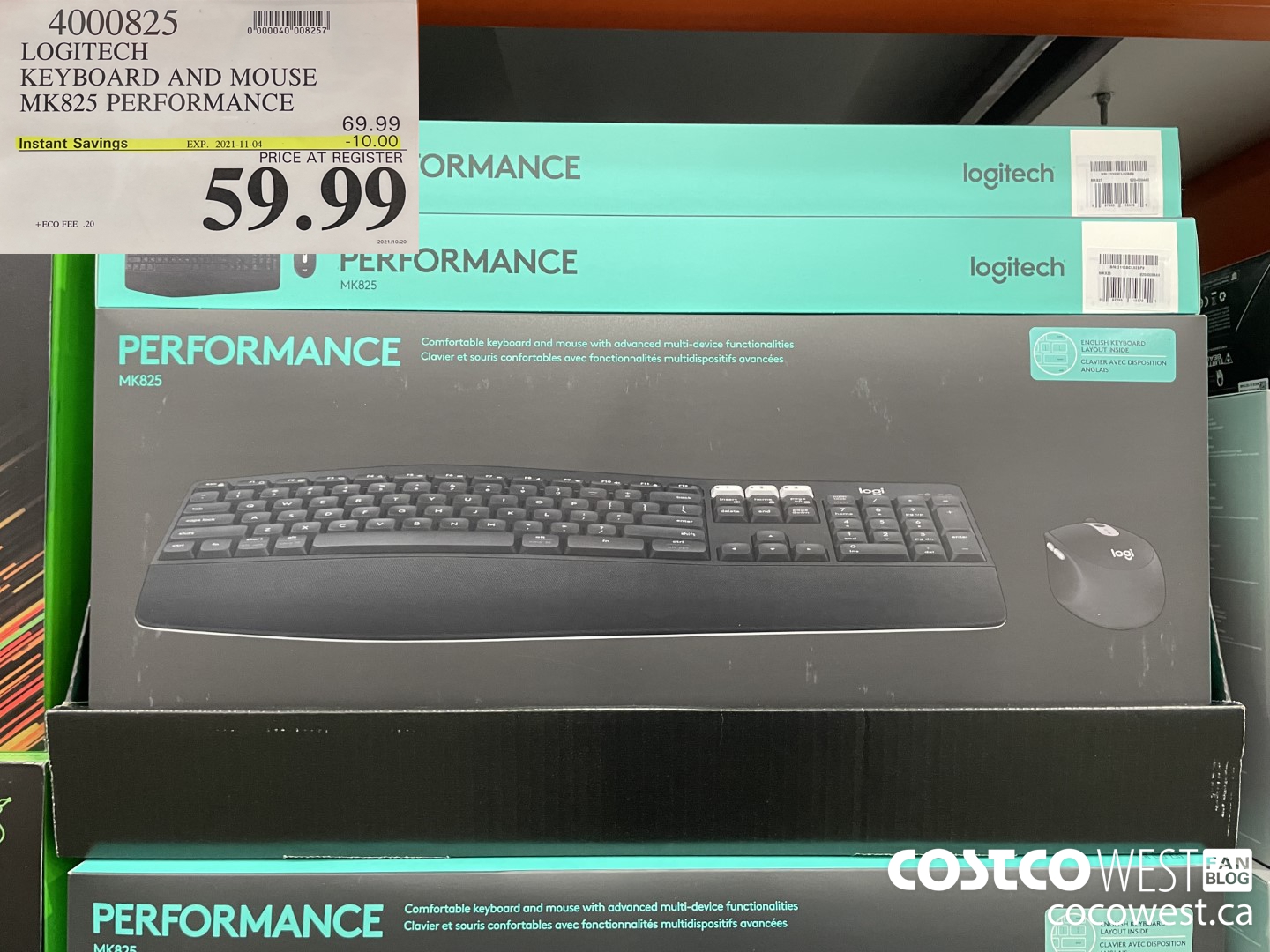The image depicts a store shelf displaying Logitech Keyboard and Mouse MK825 Performance sets. On the top left-hand side, there is a sign with the product code "4000825," beside the product name "Logitech Keyboard and Mouse MK825 Performance." To the right of this sign is a barcode and the price details. The original price is listed as $69.99, but there is an instant savings offer of $10, reducing the price at the register to $59.99. These savings details are highlighted in yellow.

In the foreground, a boxed set of the Logitech Keyboard and Mouse is placed upright, clearly displaying the product image on the front of the packaging. Behind this box, two additional boxes are positioned vertically, showing their backside. The boxes are secured within a larger container on the shelf, presumably to keep them from falling.

At the bottom right-hand corner of the image is a watermark with the text "Costco West Fanblog, CocoaWest.ca."